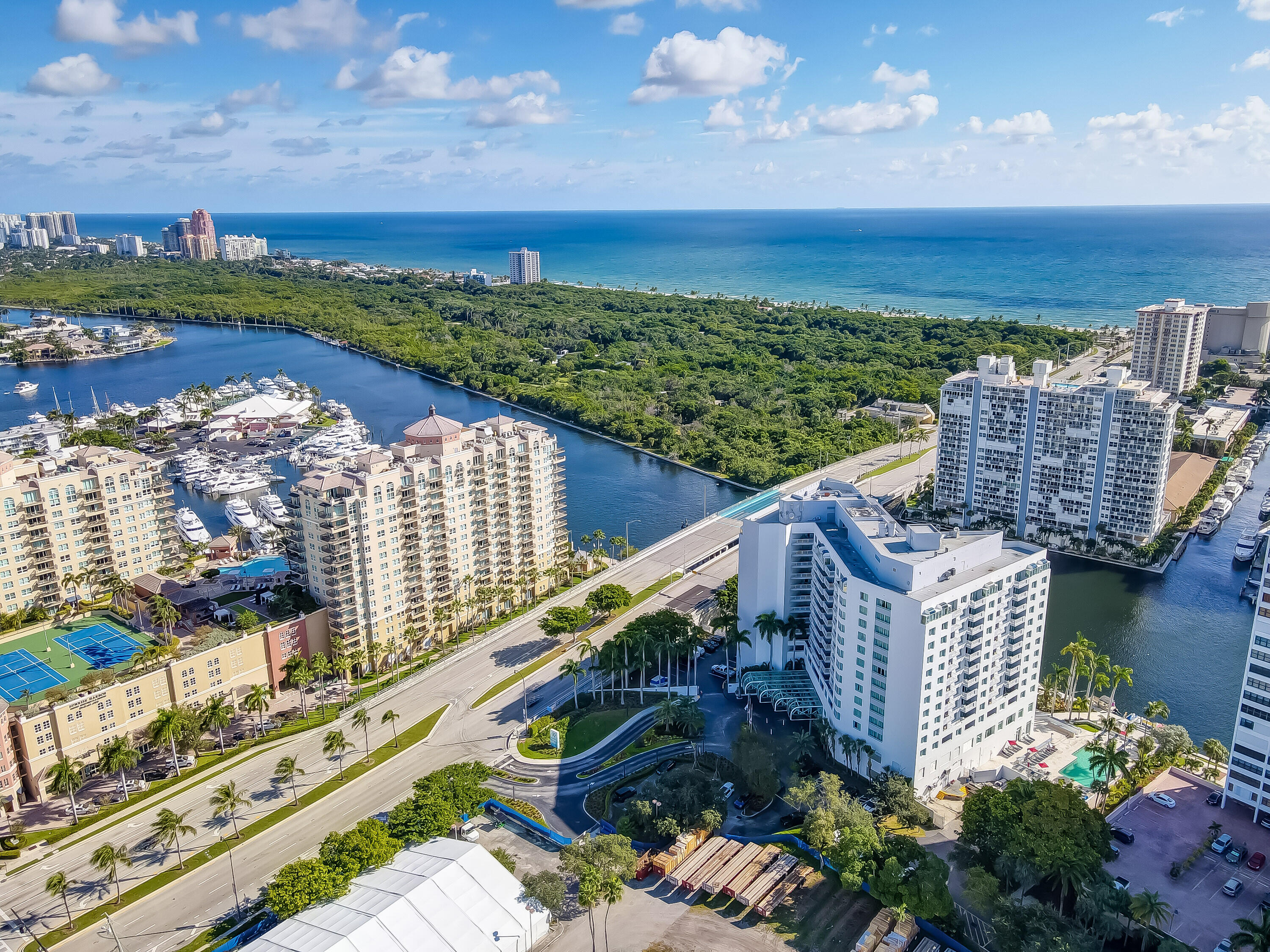This aerial photograph, likely taken from a helicopter, captures a vibrant coastal city with stunning detail. The central feature is a major highway flanked by tall, white condominium buildings adorned with numerous windows. On either side of the highway, channels of water host a myriad of boats, with a bridge allowing cars to traverse these waterways. Surrounding the highway are lush green areas filled with towering palm trees, and a noticeable tennis court adds to the recreational vibe. In the background, tall buildings rise behind patches of dense greenery. The scene extends to a sprawling ocean, over which a bright blue sky dotted with fluffy white clouds stretches. The overall landscape suggests a bustling, picturesque area, reminiscent of Florida's coastal cities.